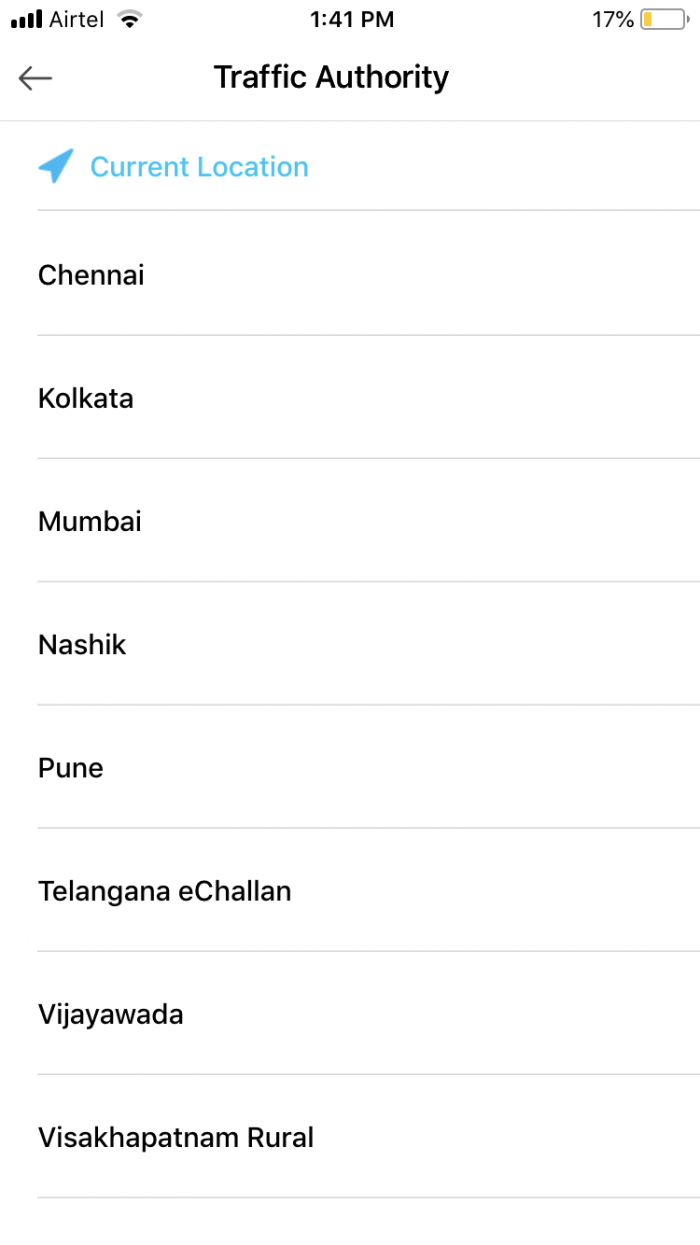A detailed image caption for the provided description:

"A screenshot of a cell phone display with a predominantly white background and black text, segmented by lines. The screen lacks a border around the edges. The phone's status bar at the top shows the Wi-Fi symbol and signal bars next to the carrier name 'Airtel' on the left side. The current time, '1:41 PM,' is centered at the top, and the battery indicator on the right shows '17%' with a small yellow mark. Below the time, the header reads 'Traffic Authority.' A line below this header indicates 'Current Location' marked in blue, accompanied by a small arrow pointing toward the northeast. The main body of the screen lists several cities and regions, presumably in India, in the following order: Chennai, Kolkata, Mumbai, Nashik, Pune, Telangana, Echelon, Vijayawada, and Visakhapatnam Rural."